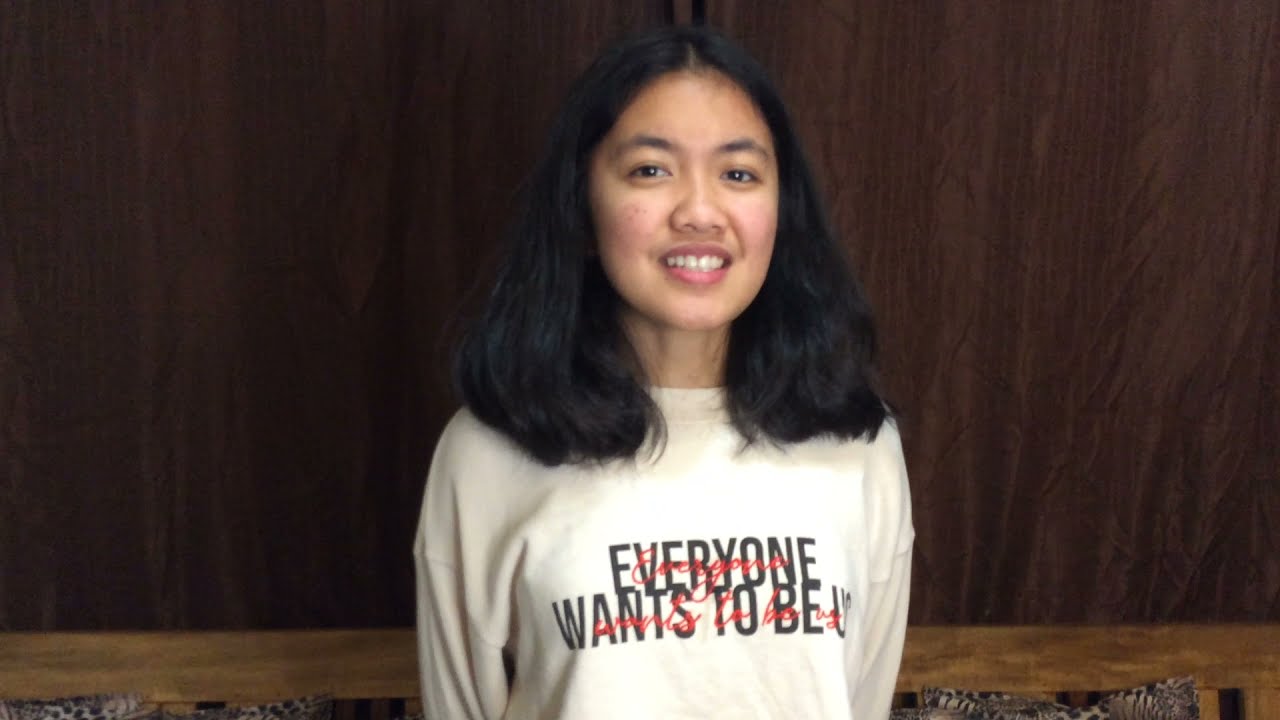The photograph depicts a young Asian woman, likely in her late teens to early 20s, standing inside a house or building against a wooden wall. There's a bench along the bottom of the image, and the woman is framed from her upper belly upwards. Despite the poor quality of the image, which is blurry and out of focus, certain details are discernible. She has long black hair that falls a bit past her shoulders and is parted in the middle. A small, shy smile reveals her teeth, and her brown eyes are slightly lit despite the insufficient lighting. She is dressed in a slightly off-white sweatshirt adorned with the black text "everyone wants to be you," where 'you' is written as 'U'. Over this text, there is some less legible red cursive writing. Her cheeks have a touch of red, as if she’s lightly blushing. Her arms are positioned behind her back, further emphasizing her modest demeanor.